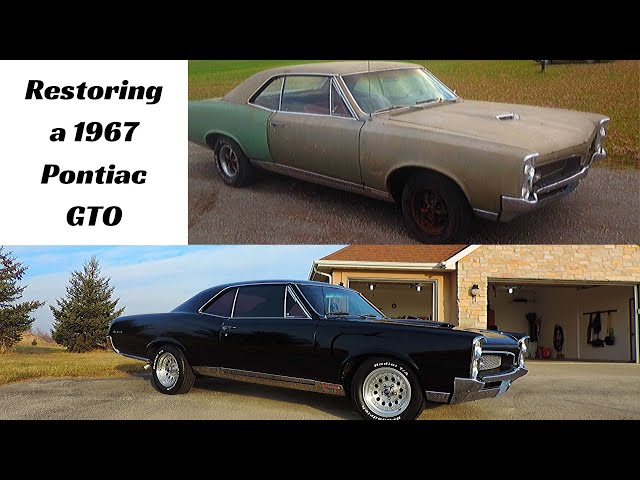In the image, there is a before-and-after comparison of a 1967 Pontiac GTO restoration. The image is framed with thick black borders at the top and bottom. In the top left corner, black text on a white background reads, "Restoring a 1967 Pontiac GTO." 

The top half of the image showcases the car pre-restoration. This version of the Pontiac GTO is depicted with a dull, two-tone finish, featuring a mostly tan body with the rear panel in a mint green, visibly dented and flawed. The car sits on an asphalt pathway next to a green lawn, with its front rims missing and the tires looking old and worn.

In the bottom half, the restored GTO is shown in a shiny black finish with new, identical shiny chrome wheels. This version is parked in front of a beige house with a brown roof, an open garage door, and blue sky and pine trees in the background. The transformation highlights the car's revitalized aesthetic, with polished chrome and a fresh, glossy paint job.